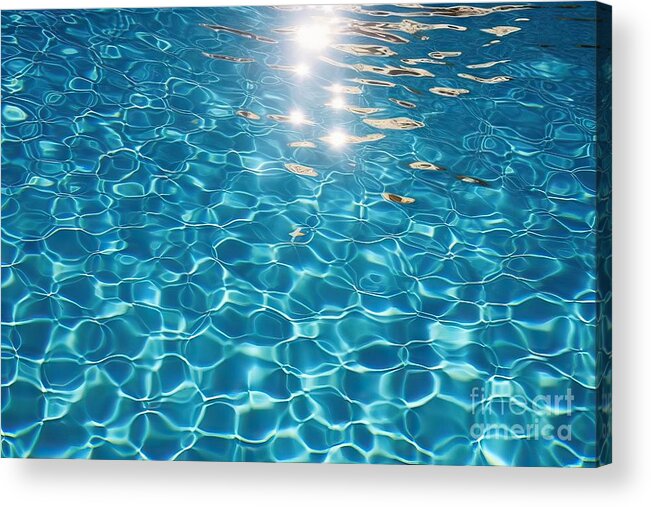This is an incredibly detailed and realistic painting, executed on a canvas in a landscape orientation, that portrays rippling water, which could be from a pool or a natural body like the ocean. The clear blue water features various shades of blue, green, and even metallic silver tones, capturing both darker and lighter hues. The light reflecting off the water creates a mesmerizing pattern of overlapping and wobbly circles, giving the impression of shimmering, almost like electricity. A bright, white glare from the sun is prominently visible in the upper half of the painting, with additional reflections contributing to the water's metallic look, especially near the top center and right. On the bottom right-hand corner of the canvas, there is a light white watermark that reads "Fine Art" on the first line and "America" on the second line, all in lowercase letters.